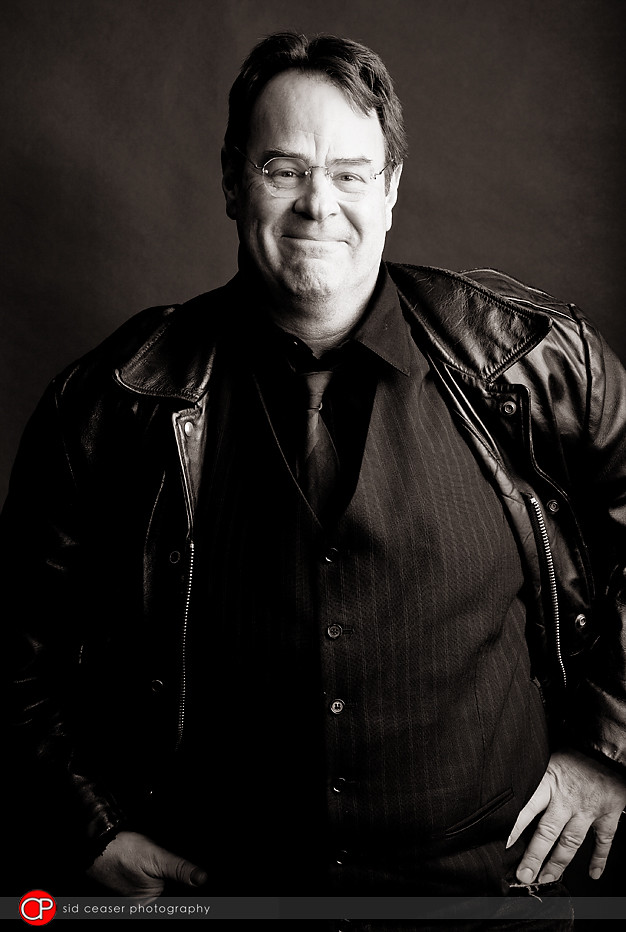This black and white photograph captures Dan Aykroyd, known for his role in Ghostbusters and Saturday Night Live, in what appears to be a professional studio shot. He is portrayed from the waist up, standing against a gradient background that transitions from dark gray at the bottom to a lighter shade near the top. Aykroyd, now middle-aged with short, dark brown hair parted in the middle, wears wire-rim glasses and is smiling gently at the camera. His attire includes a black leather jacket worn over a black pin-striped vest, a black dress shirt, and a dark tie. With his arms bent at the elbows and hands placed confidently on his hips, Aykroyd exudes a charismatic presence. The photograph features a logo in the lower left corner depicting a red circle with the white letters "CP" inside, accompanied by the text "Sid Caesar Photography" in white, which is partially overlaid on a transparent gray bar.